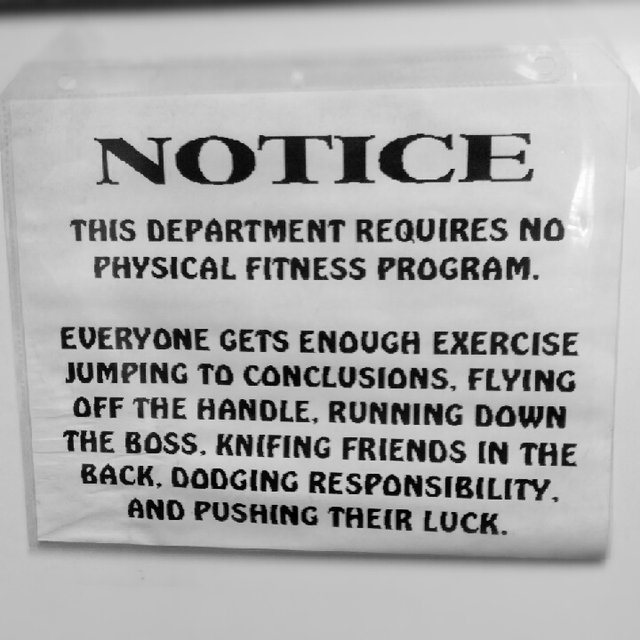This image depicts a photograph of a humorous notice hanging on a plain, stark white wall, likely covered in plastic wrap, giving it a shiny texture. The sign, which appears somewhat aged, features bold, black lettering at the top that reads "NOTICE." Below this prominent heading, in smaller bold black print, it humorously states, "This department requires no physical fitness program." It goes on to explain that everyone already gets enough exercise by "jumping to conclusions, flying off the handle, running down the boss, knifing friends in the back, dodging responsibility, and pushing their luck." The combination of sharp wit and sarcastic commentary is the focal point of this slightly worn yet visually striking notice.